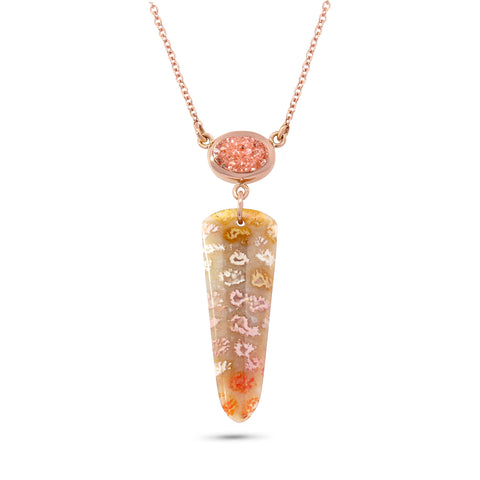This is an up-close photograph of a necklace displayed on a transparent or white background, possibly for a jewelry catalog or store display. The necklace features a delicate gold chain attached to an oval-shaped pendant with a salmon-colored, pink rhinestone encased in a golden rim. Below the oval pendant, a long, faceted, tapered agate stone dangles, resembling a spear point or wand. The agate stone is intricately colored with a variety of hues including yellowish-brown, beige, light pink, orange, white, and dark red, featuring ribbony, rounded patterns and white inclusions. The entire structure is connected through gold hooks and loops, enhancing its ornate and fancy appearance. The combination of the sparkling pink gemstone and the richly colored agate makes it suitable for both casual and dressy occasions.